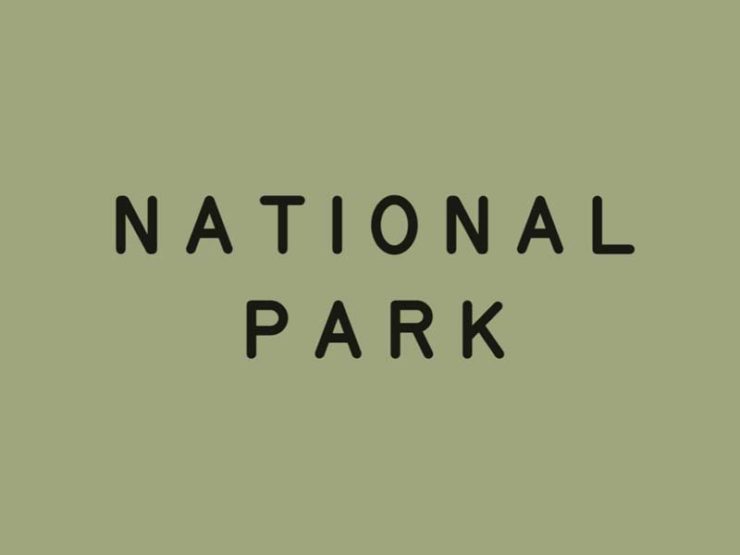The image showcases a plain, computer-generated design that appears to be a template for a potential sign. It features a solid, medium olive-green background without any borders, giving it a clean and simple look. Centered in the middle of this background are the words "National Park," written in all capital black letters, each word stacked vertically with "National" on top and "Park" directly below it. The text is somewhat spaced apart, utilizing a straightforward and easy-to-read font that provides clarity and readability. This minimalist design contains no additional images, references, or websites, emphasizing the text against the solid backdrop.